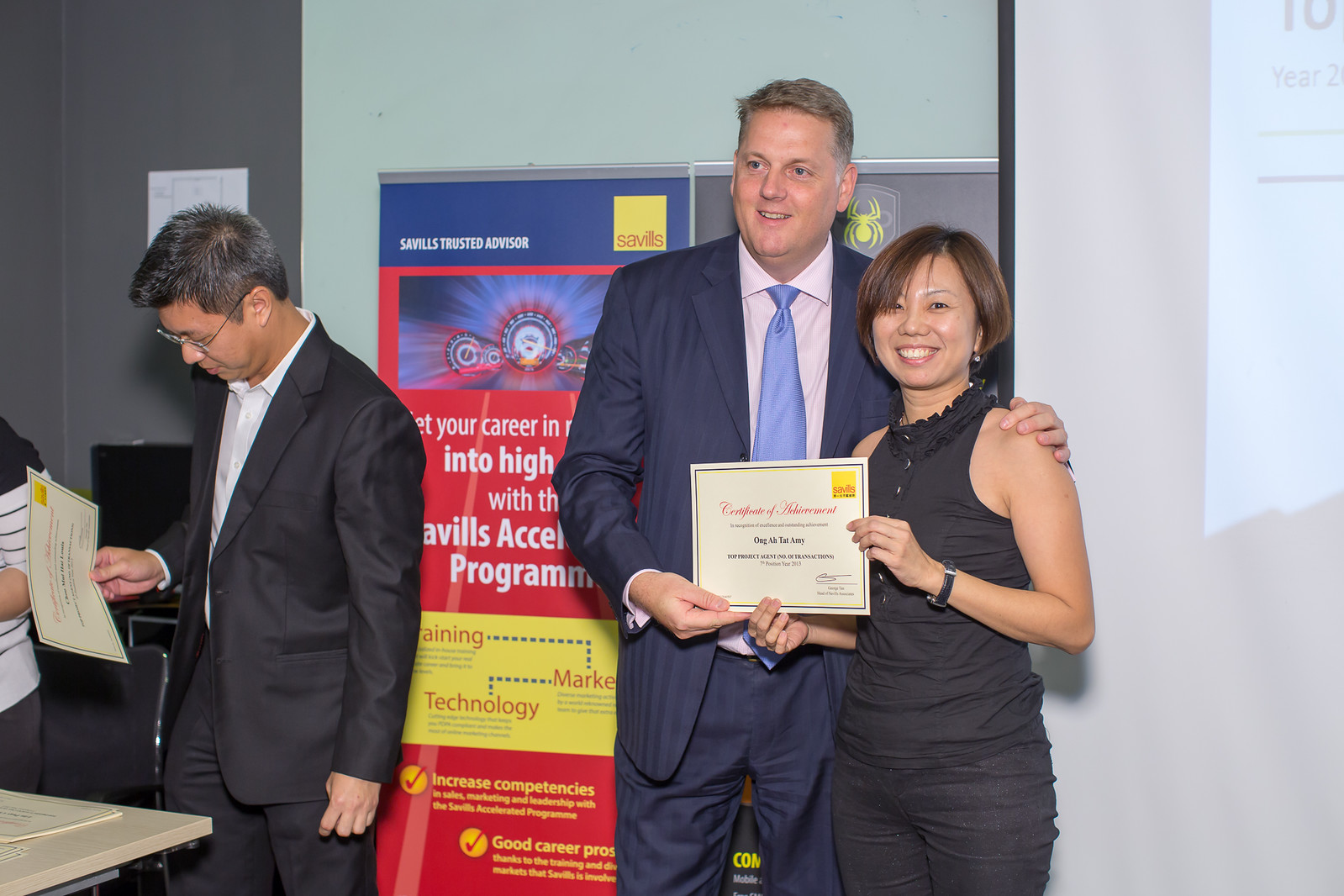In this detailed photograph, three individuals are captured in a significant moment likely set during a graduation or an award ceremony. The background is dominated by a gray and white wall adorned with a red and yellow advertisement poster promoting careers in training, technology, and marketing. On the left side stands an older Asian man with graying black hair, glasses, and a black suit over a white shirt. He is intently looking down at a paper, presumably a certificate, that he holds in his right hand above a table.

To his right, centrally located in the frame, stand a white man and an Asian woman. The man, clad in a blue suit with matching dress pants, a blue striped tie, and a pinkish shirt, has his arm affectionately draped over the woman's shoulder. The woman, distinguished by her short brown hair and bright smile, is dressed in a stylish black sleeveless top, a black necklace, and black pants. Together, they hold a certificate, which the man appears to be presenting to the woman. She looks elated, beaming with happiness at the recognition. The atmosphere and context suggest this is a celebratory event, commemorating achievements and milestones.